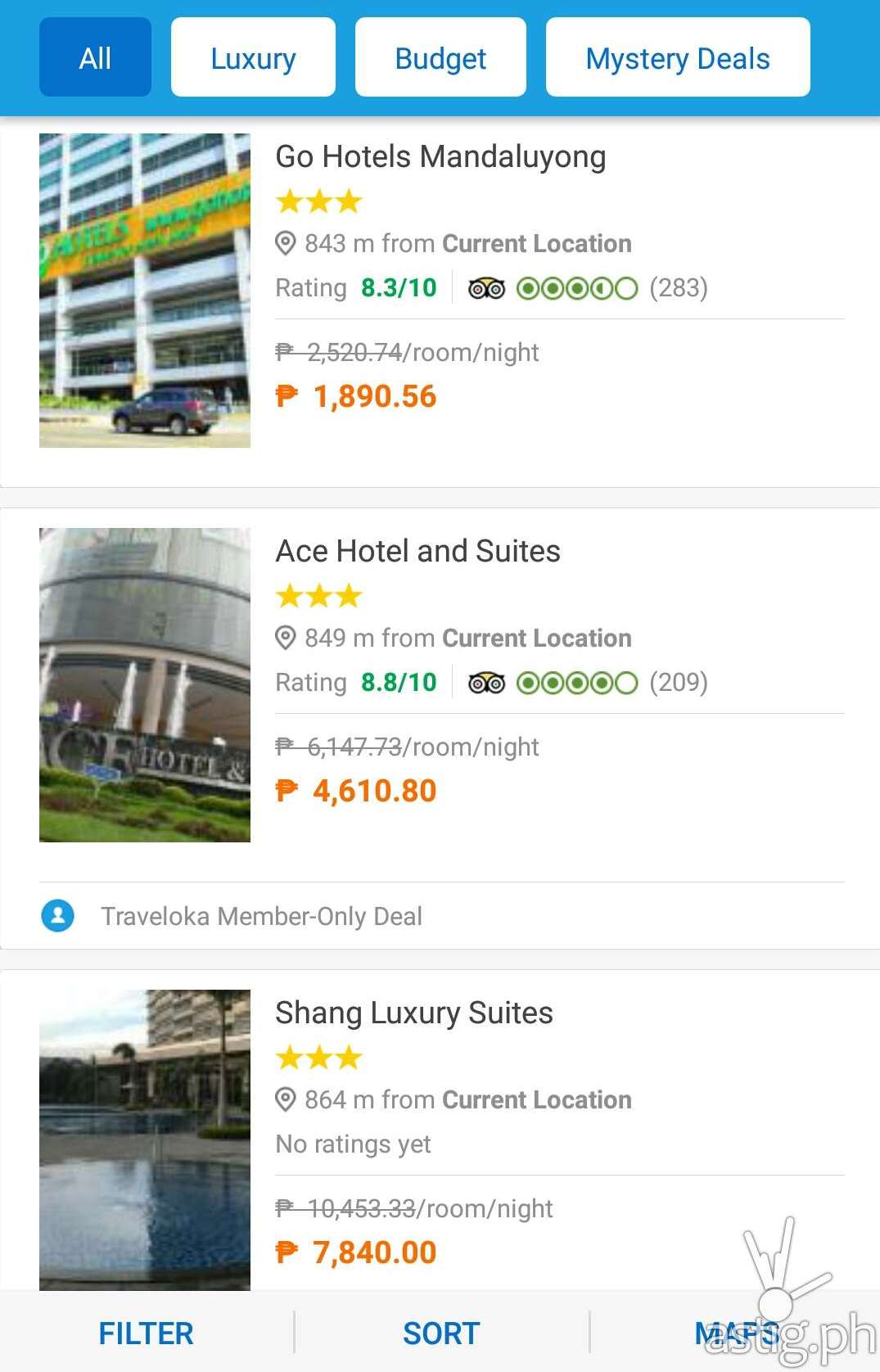Here is a detailed and cleaned-up descriptive caption for the image:

---

This screenshot features a user interface with a sky blue header running across the top. Embedded within the header are four square or rectangular buttons. The first button on the left is dark blue and labeled "All" in white text. Next to it, there is an aqua blue button labeled "Luxury". The third button, also in aqua blue, is labeled "Budget", and the final button on the right, again in aqua blue, is labeled "Mystery Deals".

Beneath these buttons, the screen displays search results, each accompanied by a photograph of a building on the left. The first result displays "Go Hotels, Mandaluyong" in bold black text. Below this, there are three yellow stars, followed by a small map icon and the distance "843M from current location". A user rating is also shown below this information.

The second result is for "Ace Hotel and Suites", which also has three yellow stars and is "849 miles from current location".

The third listing is for "Shang Luxury Suites", also rated with three stars and "864M from current location".

At the very bottom of the screen are three buttons with a gray background, separated by vertical light gray lines. The buttons are labeled in aqua blue text from left to right as "Filter", "Sort", and "Map".

---